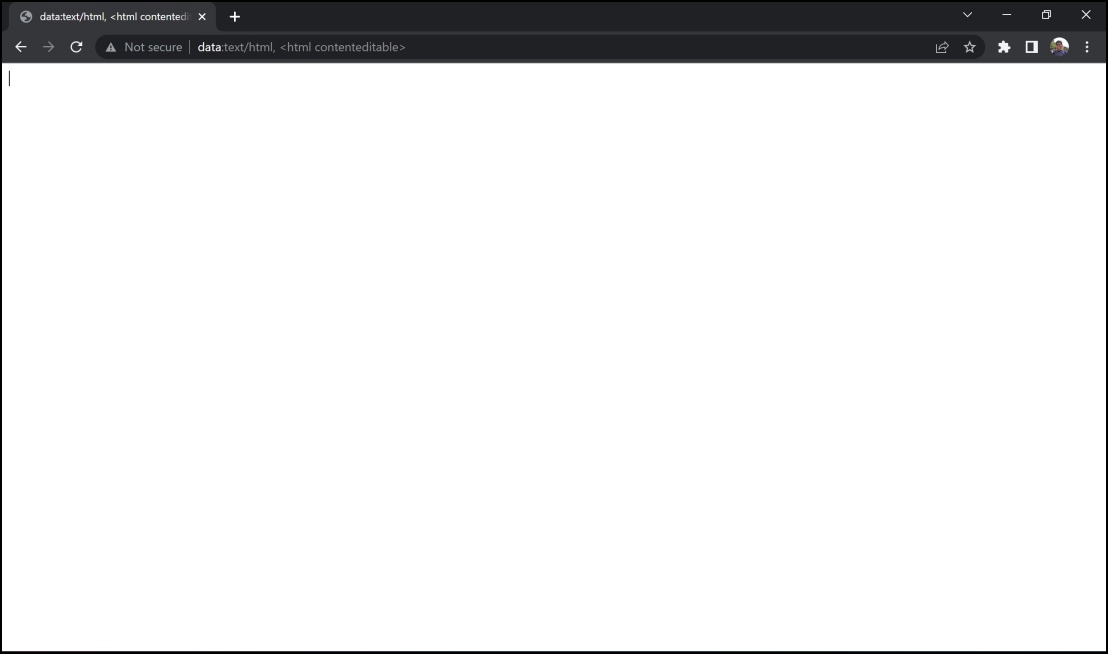The image captures a screenshot of a laptop or computer displaying a specific webpage. The browser's top bar is a darker gray, showcasing a tab that is currently open. This tab displays a white icon of the Earth and the text "data.txt/html" in white. To the left of the text is a less-than symbol (<), indicating HTML content. An 'x' symbol is available for closing the tab.

Just below the top bar are the navigation buttons for moving back and forth between pages, a circular arrow icon for refreshing the page, and the address bar. In the address bar, there is an exclamation mark within a triangle, followed by the text "Not Secure" in gray. The address itself reads "data:text/html" with HTML content indicated by less-than and greater-than symbols surrounding the word "contended table." To the extreme right of the address bar, there is a star icon and a white puzzle piece representing browser extensions. There's also a small, circular profile picture that is difficult to discern but appears to show a Caucasian individual wearing a gray shirt.

The main body of the webpage is entirely blank, filled only with white space.